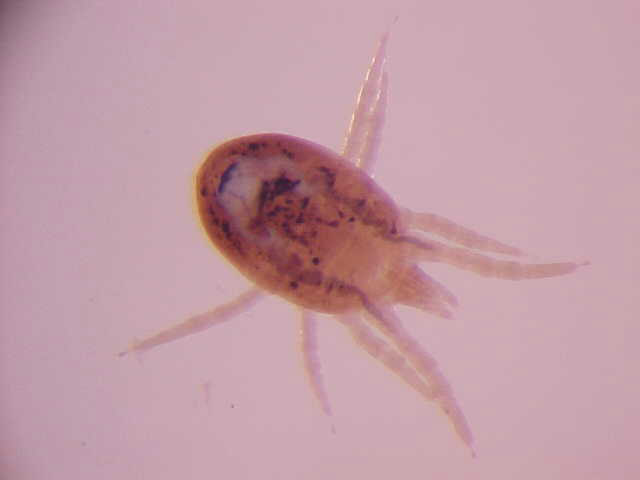The image is a close-up, microscopic view of a tick or similar mite-like creature. The rectangular photograph measures about four to five inches wide and three to four inches high. The backdrop is a light pink shade, which transitions to dark, almost black tones in the upper left and lower left corners, suggesting the effect of a light shining through translucent paper.

The tick itself, centrally positioned, is oriented with its oval-shaped body pointed towards the upper left corner. The body is light brown with scattered dark spots and amber to reddish undertones. It features eight elongated, tube-like legs which are mostly white and end in pointed tips. The legs are divided into pairs with four thrust forward, resembling pincers, and four splaying to the sides.

Light surrounds the tick, enhancing its partially transparent sections. The body includes some darker areas in the center. A small, tail-like extension protrudes from its back end. The specific lighting and microscopic detail reveal even minute features, adding to the intricate depiction of this tiny arachnid-like creature.